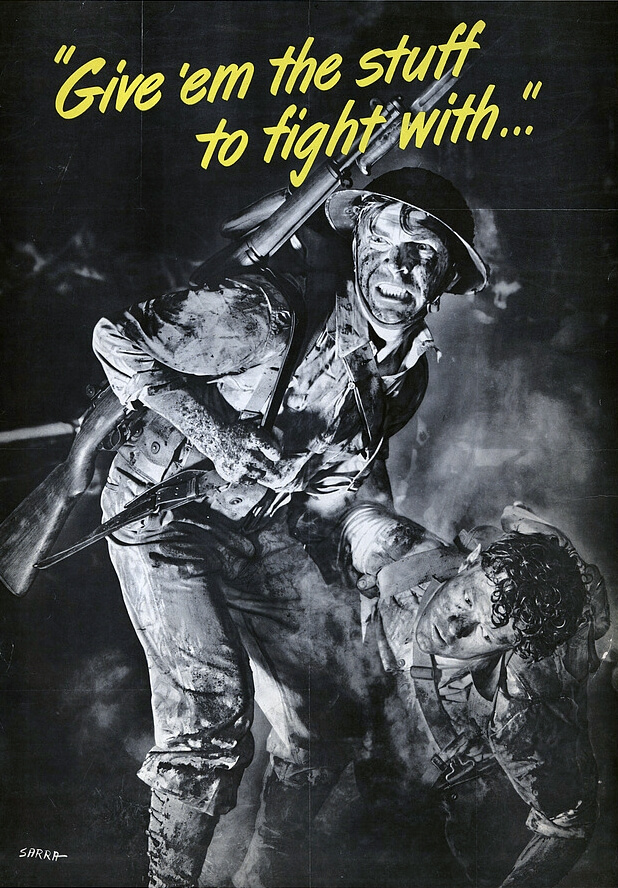The image is a black-and-white photograph or poster set against a dark background, likely from an old war movie or an advertisement, depicting a distressing scene from World War I. Central to the image are two soldiers in uniform, highlighted by a light source from the left. The standing soldier, donned in a typical World War I tin helmet, a rifle secured over his shoulder with a strap, grimaces as he looks to his left. He wears short breeches, gaiters, and sleeves that fall just below his elbows, and his muddy, straggly hair indicates the harsh conditions. His arm supports his comrade, who is crouched or kneeling with one arm on the ground, looking down with a pained expression. The second soldier, helmetless, shares a grimy appearance, and his curly hair adds to the scene’s raw authenticity. Both soldiers' faces and clothing are marked by dirt and fatigue, with fog or smoke subtly rising in the background, enhancing the overall tension and distress. At the top of the image, in striking yellow text, the caption reads, “Give them the stuff to fight with,” suggesting an appeal for support or provisions for the soldiers. At the bottom left, a signature reads “sarin—,” emphasizing the artistic or historical significance of the piece.